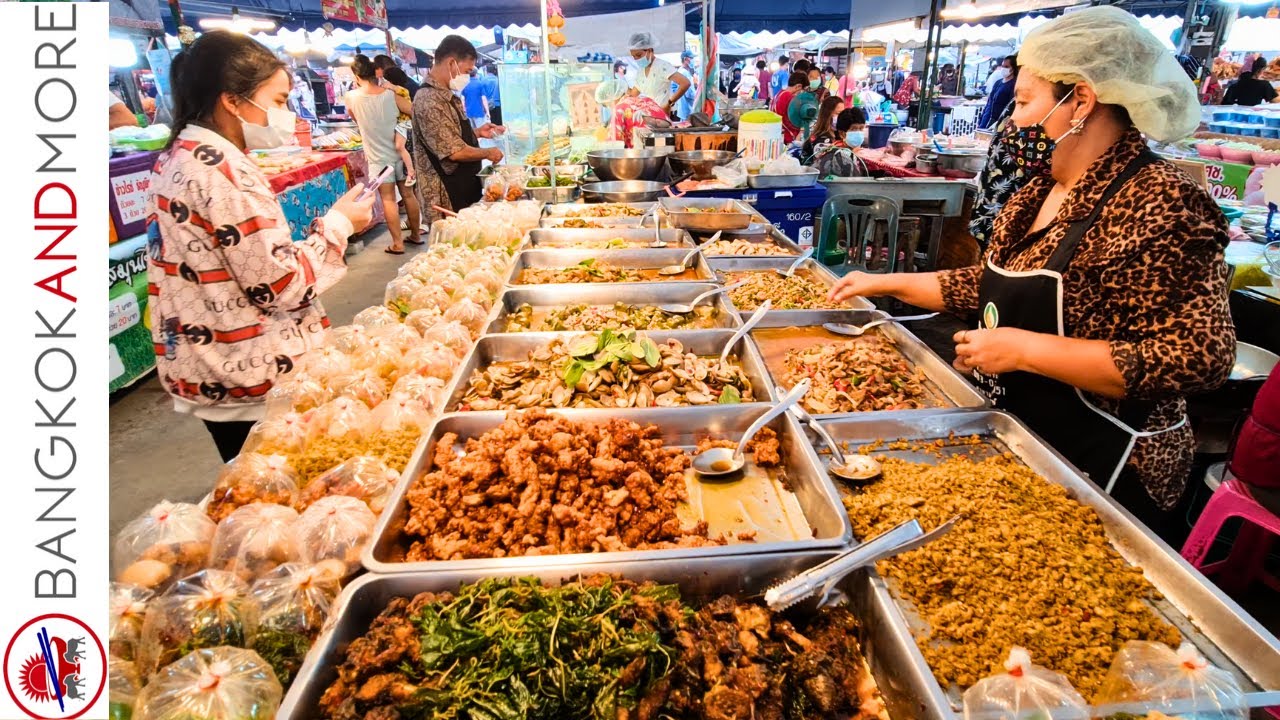The photograph depicts a bustling indoor market or buffet setup featuring an array of food items meticulously arranged in stainless steel warming trays spanning about 15 feet in three neat rows. The scene is vibrant with various colors including light brown, green, black, orange, yellow, light blue, dark blue, and off-white, suggesting a diverse selection of foods such as fried meats, vegetables, and rice.

In the foreground, on the right side of the image, a woman wearing a cheetah print top, a black apron, and a hairnet is serving food. She also sports a distinctive black surgical mask adorned with multicolored patterns. Directly opposite her, on the left, stands a customer wearing a white shirt with red or orange stripes and a white surgical mask. She appears to be making her selection from the assortment of dishes.

Further back, other people can be seen, including a lady on the left holding a child and another girl with a phone, possibly intending to purchase food. The atmosphere is lively with numerous customers and sellers interacting across the market space. There are additional tables in the background covered with red tablecloths where people are seated, most wearing masks, indicative of health precautions being observed.

Notably, the left side of the image features vertical text reading "Bangkok and More," hinting at the possible cultural or thematic motif of the market. The photograph captures the indoor ambiance of the setting in broad daylight, providing a glimpse into the dynamic and colorful environment of this food market.